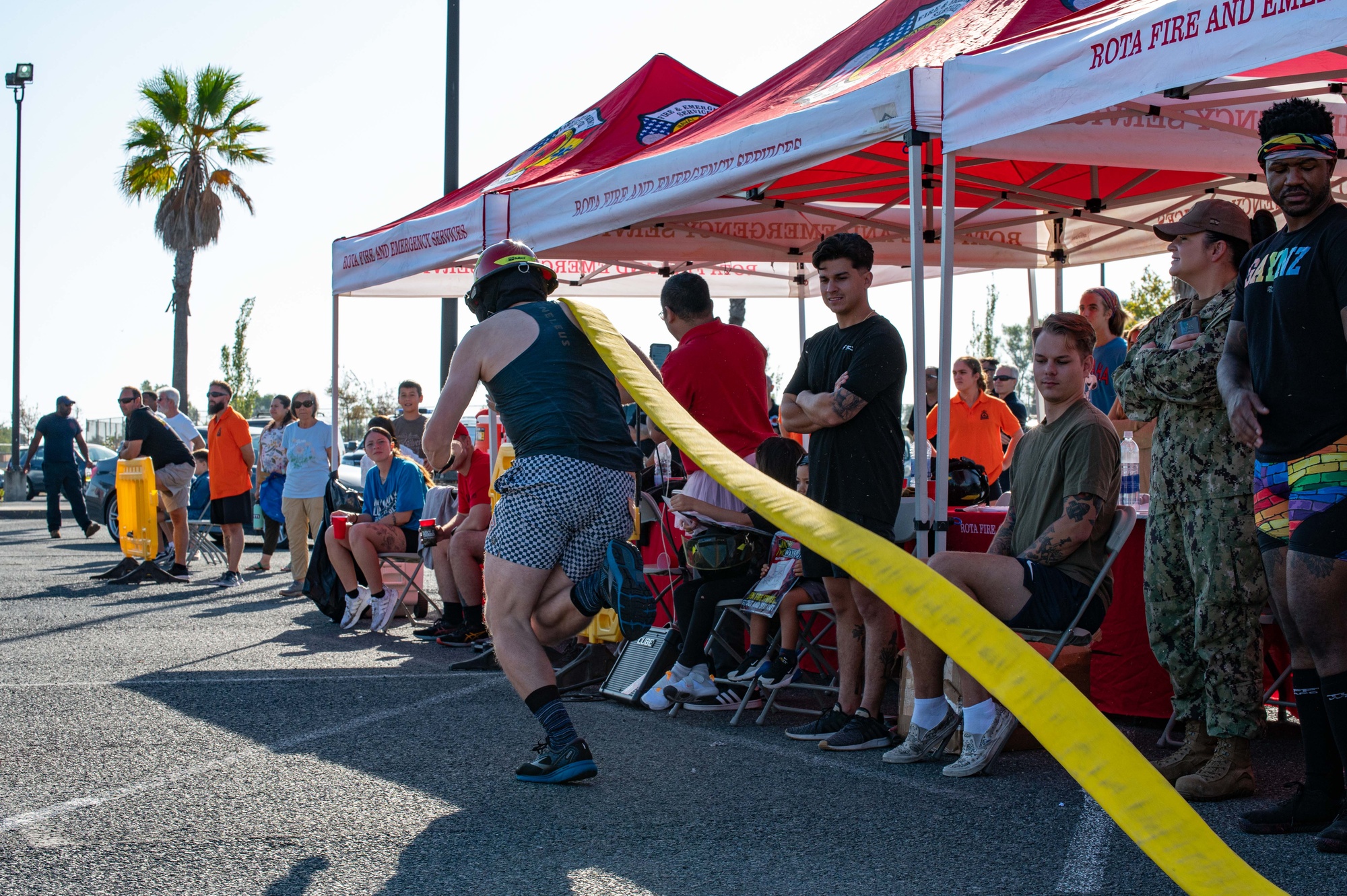Several red and white event tents are set up in a parking lot, emblazoned with the text "Road of Fire, Fire and Emergency Services." The scene is bustling with spectators, a mix of people standing and sitting on white chairs, many with their arms crossed, shaded from the sunny, albeit slightly overcast sky. A notable figure on the right is a woman in Army fatigues, adding a military presence to the gathering. A palm tree in the background hints at a warm, southern setting. The main focus of the event appears to be a man running with a long yellow fireman's hose slung over his right shoulder. He is dressed in black and white checkered shorts, long black socks, and a black tank top. His fire helmet and rapid pace suggest a competitive nature to the proceedings. Among the diverse and colorful outfits of the crowd, one man leans on an orange box, while another, in very colorful shorts and a headband, stands out. All eyes are on the runner, eagerly watching his performance.